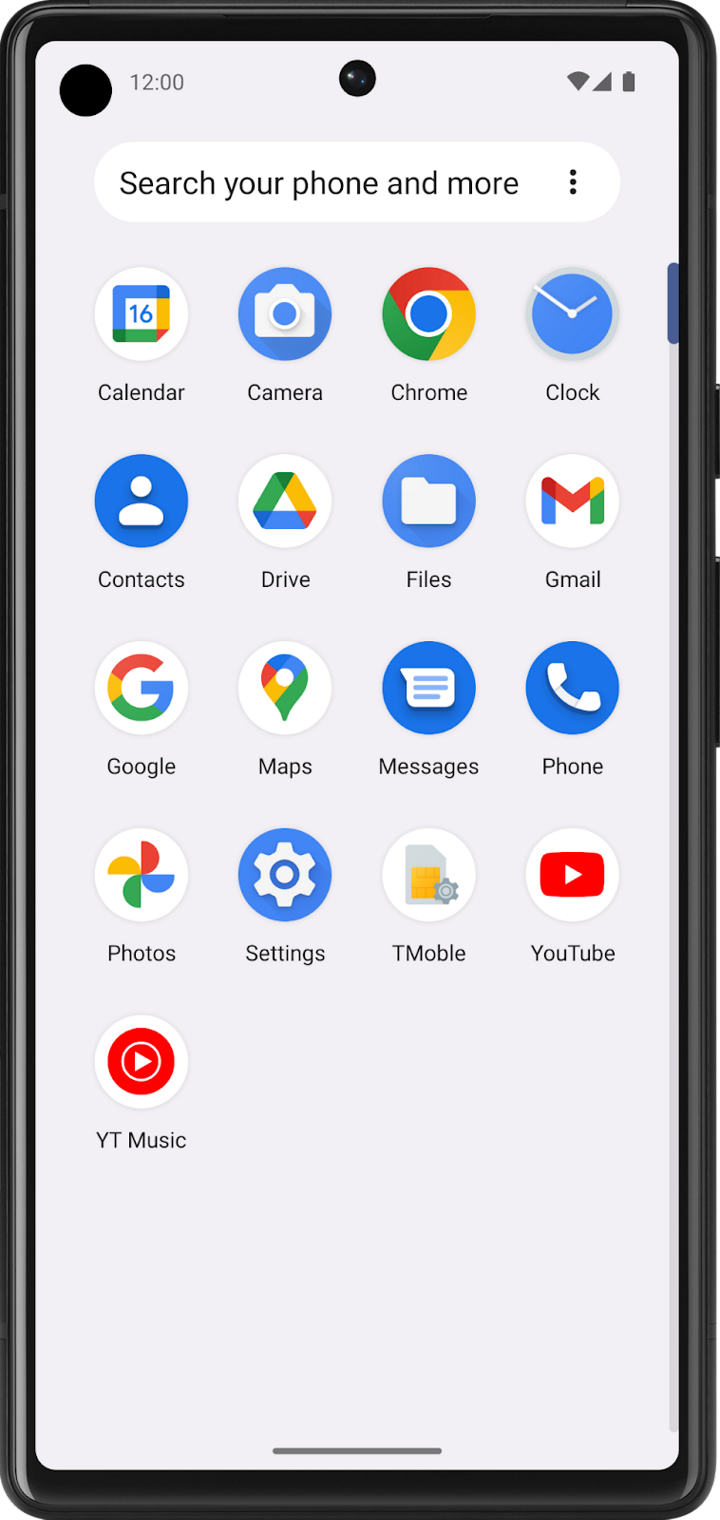A detailed screenshot of an Android device's home screen, possibly an LG phone, based on its shape and design. At the top left corner, the time displays "12:00." Centrally located at the top edge of the screen is a small camera pinhole, flanked on the right by the Wi-Fi, mobile cellular, and battery icons, indicating device status. Just below these indicators is a pill-shaped search bar with three vertically aligned dots to the right, signifying settings options.

The main screen showcases several app icons organized in rows. The first row contains "Calendar," "Camera," "Chrome," and "Clock" apps. The second row features "Contacts," "Drive," "Files," and "Gmail." On the third row are the "Google," "Maps," "Messages," and "Phone" apps. The fourth row displays "Photos," "Settings," "T-Mobile," and "YouTube." The final row includes the "YouTube Music" app.

The background is a light gray hue, while at the bottom foreground, a black lining is present, likely serving as a navigation bar, which can be tapped and swiped upwards to reveal additional pages or content.